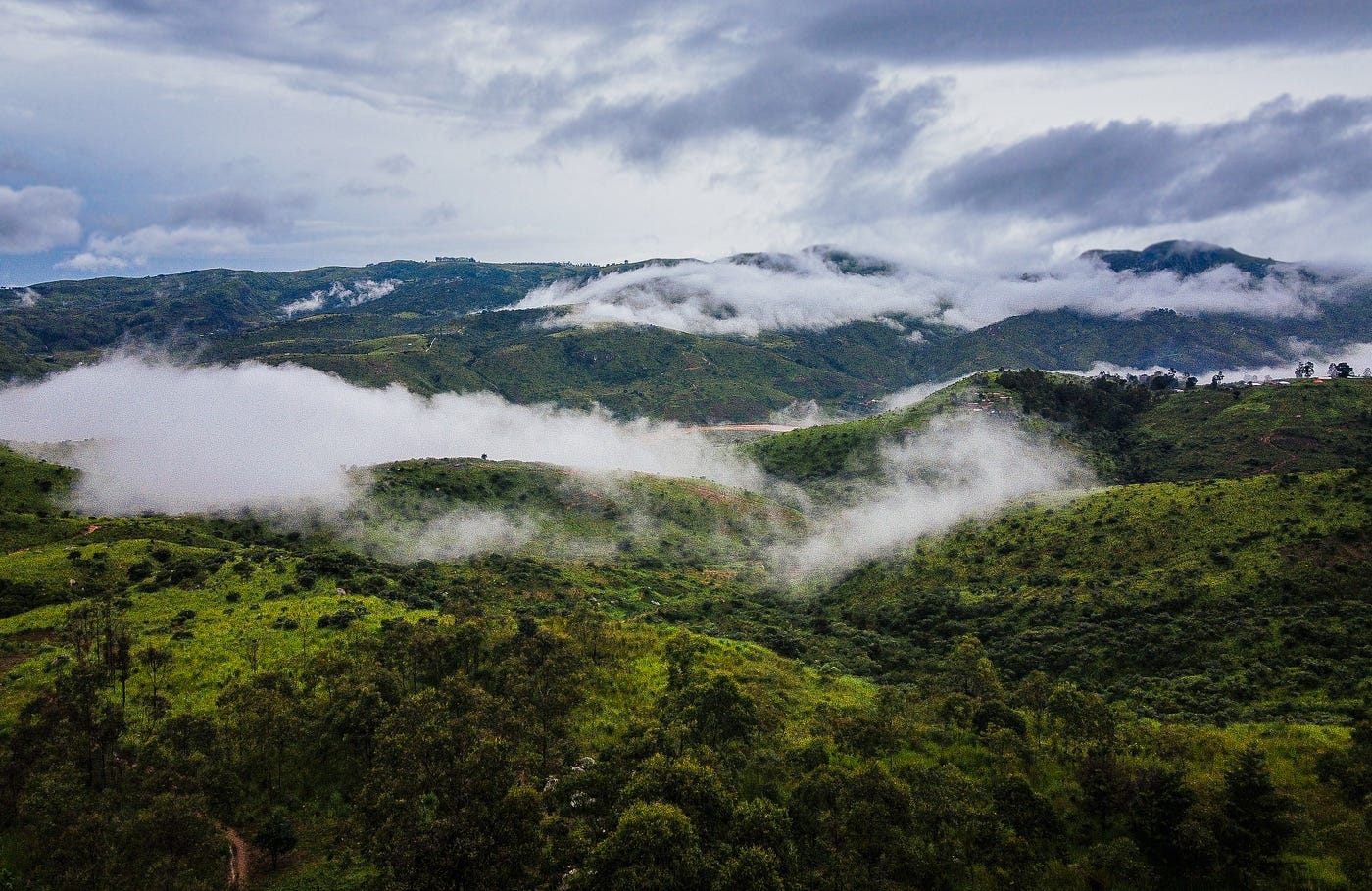The image is an aerial photograph capturing a picturesque mountainous landscape. At its center, towering mountaintops are lightly dusted with snow. A lush, green valley unfolds beneath the peaks, shrouded in rising fog. The scene is framed by rolling, hilly terrain that suggests a jungle-like environment, with the bottom left corner revealing a dirt road curving through the landscape. Birds are seen taking flight in the center of the image, adding life to the serene scene. At the middle right, several rectangular-shaped buildings stand atop a hill, seemingly isolated and without visible roads leading up to them. Above, the sky is a dramatic mix of dark bluish-gray and light blue, punctuated by bouts of white and dark clouds, enhancing the ethereal quality of this breathtaking landscape.